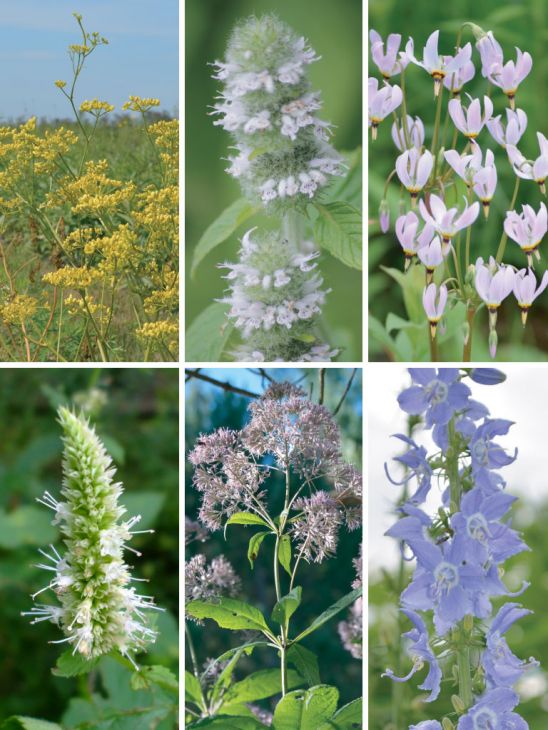This image is a collage featuring six different types of flowers, each captured in a vertically-oriented, rectangular section. The sections are uniform in size and are separated by crisp white dividers, creating a clean and organized visual. The collage is arranged with three sections on the top row and three on the bottom row.

Starting from the upper left, the first image showcases yellow flowers set against a backdrop of a blue sky and lush green foliage. The middle image on the top row features a slender green stem adorned with small, delicate white flowers. To the right, the third top-row image presents a cluster of white flowers that resemble little cups, with petals beginning to open.

In the lower left section, the image displays a green, somewhat spiky plant with white flowers concentrated towards the bottom. The middle section on the bottom row highlights thin, spindly flowers that are a mix of pink and purplish hues. Finally, the bottom right image depicts a vine-like plant, adorned with circular purplish flowers that stand out in their bloom.

Each flower is distinctly presented, allowing viewers to appreciate the uniqueness and details of each type.